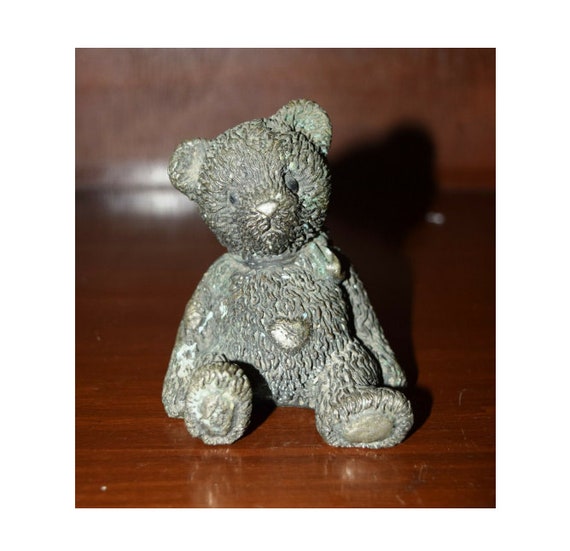The photograph showcases an old, possibly weathered, teddy bear figurine sitting on a medium reddish-brown wooden table that reflects parts of the bear and casts a shadow to the right. The bear, which appears to have rusted or patinaed over time into a grayish-brown hue with a hint of green, is designed in a cartoonish style with static limbs, typical bear ears, two black eyes, and a light gray nose. Its head is subtly cocked to the side and a small scarf adorns its neck. The arms hang down by its sides, and a heart emblem is featured on its tummy, blending into the bear's uniform patina. The background is blurred but continues the brown tone of the table. The bear is illuminated by a light source, likely a camera flash, creating a shadowed effect to the right side of the image.